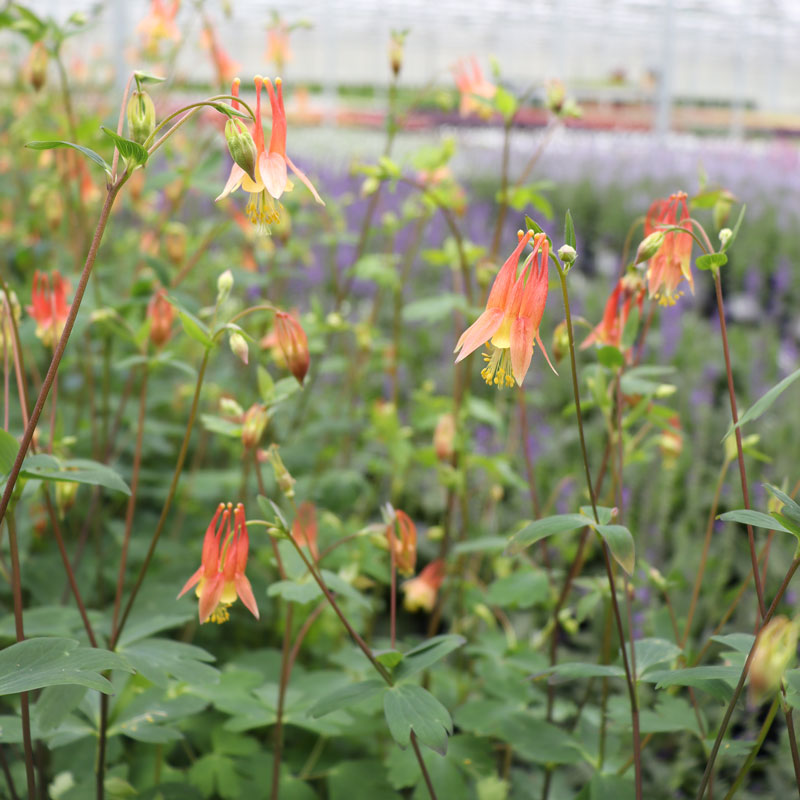This image captures a close-up view of several orange, bell-shaped flowers on long, thin stems with sparse green leaves. Each flower droops downward and features a typical 4 or 5 petal formation with prominent yellow stamens emerging from the center. Some stems remain single and undivided while others may branch once or twice. There's an abundance of these flowers, with at least 20 in view, gradually losing focus and blending into the background. Blurry but faintly visible is a greenhouse structure, suggesting the flowers might be cultivated indoors. The greenhouse and other distant flowers are indistinct, enhancing the clarity and vividness of the orange blooms in the foreground. Some stems also display budding green flowers yet to open.